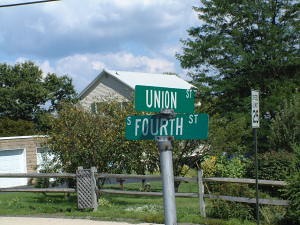This photograph captures a charming street corner in a residential neighborhood under a vibrant blue sky dotted with fluffy white clouds. Dominating the scene is a standard green street sign mounted on a galvanized metal pole; the sign facing the viewer reads "S 4th Street," and the adjacent sign, perpendicular to it, reads "Union Street," indicating the crossroad of Union and 4th Streets. Nearby, a white speed limit sign indicates a 25 mph limit. In the background, a wooden fence with concrete posts encloses a yard, adorned by greenery with bushes and a prominent tree. Visible behind the fence is a two-car garage with two white doors. Beyond the garage, a two-story house with a white roof makes its presence felt, suggesting a quiet and picturesque neighborhood setting.